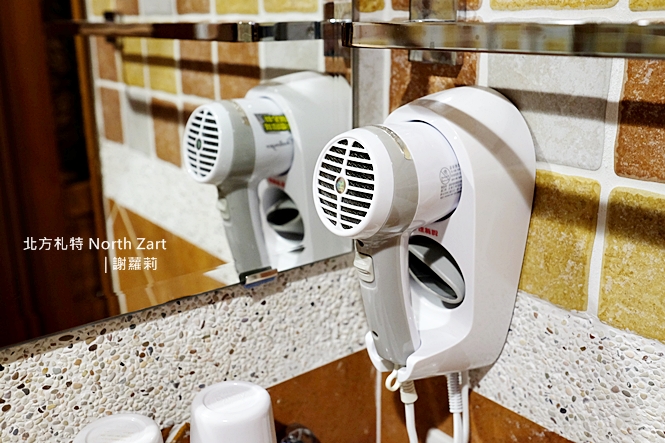This photograph depicts a small section of a hotel bathroom, focused on a wall-mounted white blow dryer with a gray handle. The blow dryer, featuring a black filter vent on its back, is affixed to a multicolored tile wall in a corner, showcasing tiles in mustard yellow and burnt orange hues. Mounted below a stainless steel towel bar, the blow dryer stands in front of a mirror, capturing both its direct view and reflection. The mirror, positioned to the right, includes a watermark with Asian characters and the words "North Zart" in English. The bottom part of the image reveals several disposable cups, suggesting the hotel setting. The lower section of the wall also displays a fine mosaic tile pattern in gray with flecks of brown and beige.